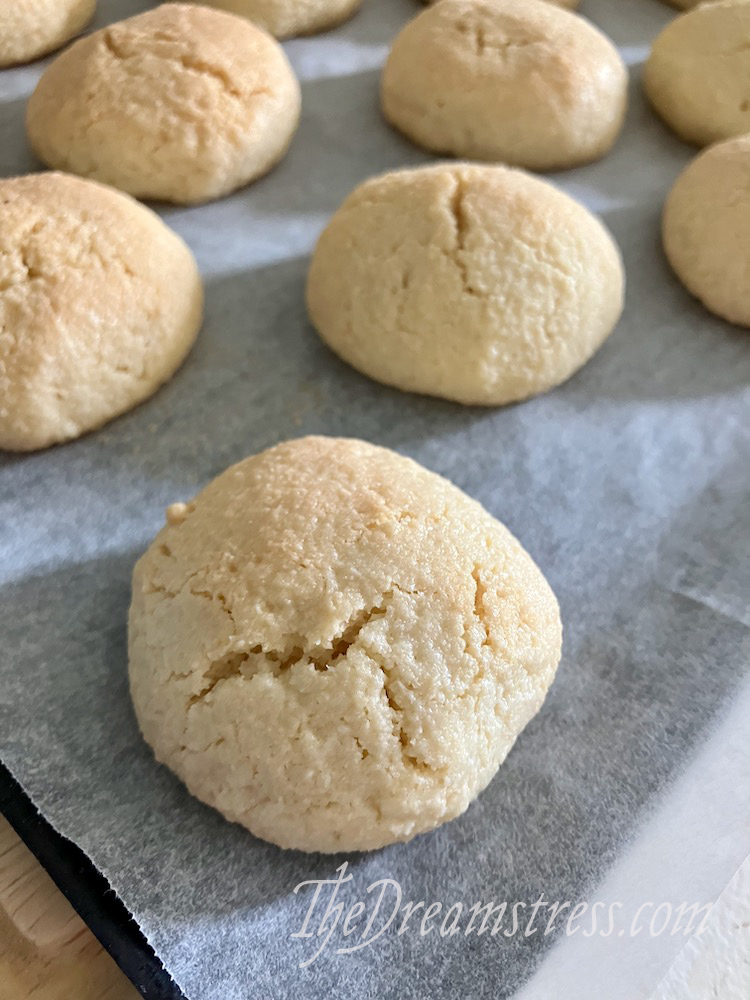This close-up, color photo features seven small, round baked goods that bear resemblance to either scones or sugar cookies. Each item is uniformly yellowish-brown and exhibits visible cracks, indicating a cake-like texture. Arranged on a piece of white parchment paper covering a black tray, these baked treats are aligned in rows. The parchment paper gives the illusion of a gray cloth beneath them. In the bottom right corner of the image, "thedreamstress.com" is elegantly written in white cursive font. The overall presentation highlights the soft, slightly sugary appearance of these delectable-looking baked items.